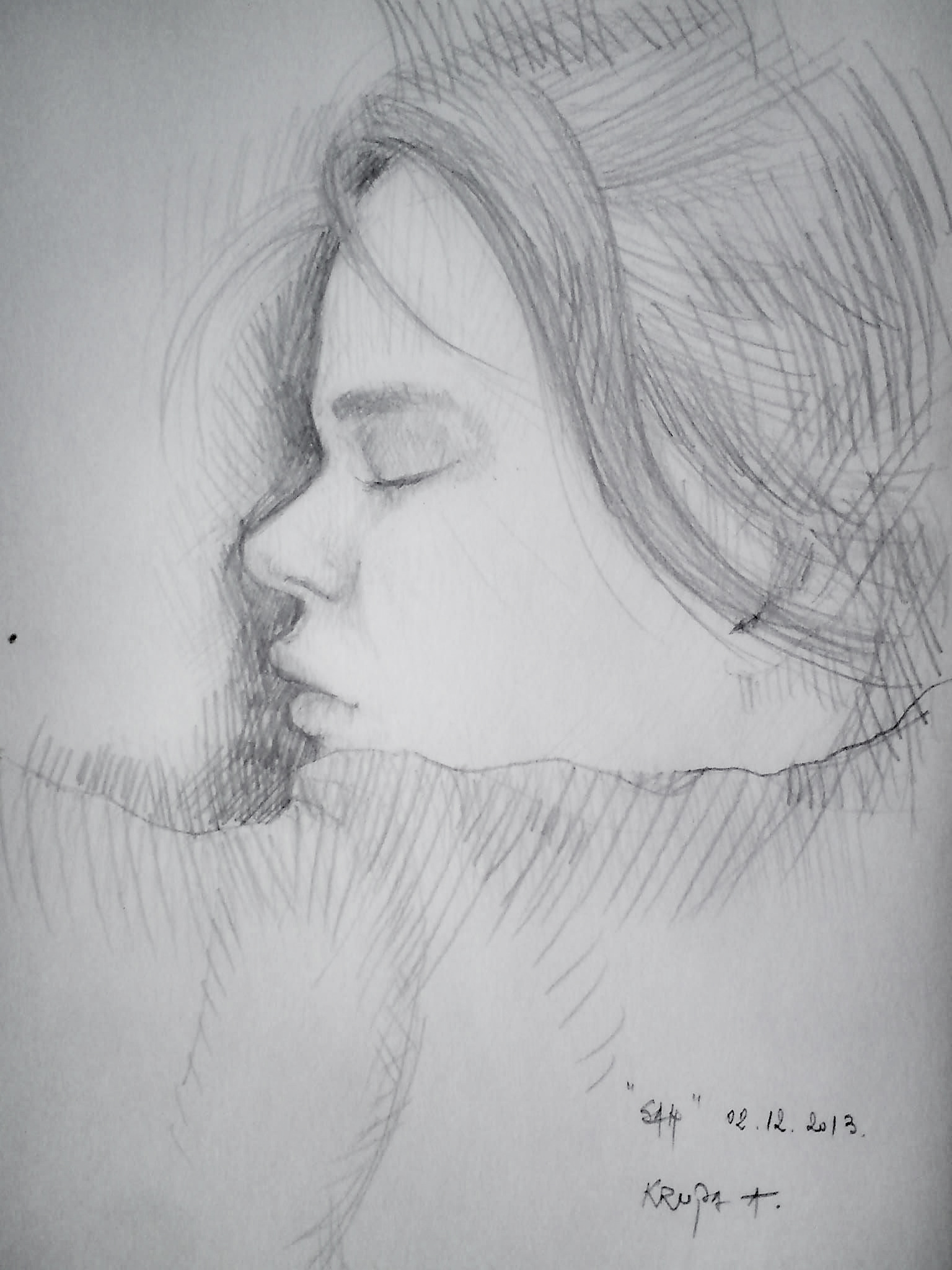This detailed, pencil-drawn sketch captures a serene and intimate scene of a woman, or perhaps a little girl, lying down. Her closed eyes and slightly parted full lips give a sense of peaceful rest. The drawing is in black and white, using varied shading and lines to create depth, particularly noticeable in the shadowed area beneath her face. She has long, cascading hair that drapes over the right side of her face, partially obscuring her pointed nose and giving a soft, messy appearance as it flows around her. The blanket pulled up to her chin conceals her neck and chin, adding to the cozy and tender atmosphere of the sketch.

The scene is a side view, with her face oriented towards the left edge of the paper. There is a signature located at the bottom right, comprising the initials "K-R-U-P-E-R-T", beneath a date inscribed as "02-12-2013". Additionally, near the top, there is an inscription in quotation marks, partially legible with letters resembling "S-A-A S-A-H". The background is lightly shaded in gray, enhancing the focus on the resting figure. The meticulous details and emotive quality of the sketch reveal the artist's skill and the tranquility of the subject.